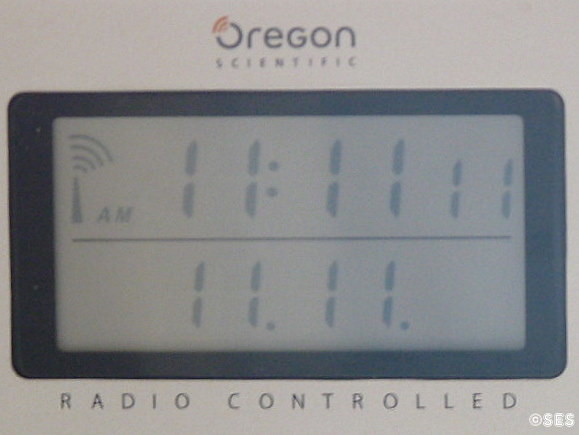The image depicts a control panel with a white background, prominently featuring the text "Oregon Scientific" at the top center in black. The 'O' in "Oregon" is uniquely marked with orange Wi-Fi-like lines radiating upwards to the left. Centrally positioned below this text, there is a rectangular display screen framed in black with a gray interior showing black numbers. On the left side of the screen, there is a depiction of an antenna emitting signal lines towards a hub, and the text "AM" in black, accompanied by the number "111111" and the sequence "11.11.11". Below this screen, the text "radio controlled" is displayed, also in black, extending from left to right. At the bottom right, the logo "SES" appears, repeated on the left side of the text along with the copyright symbol 'C'.